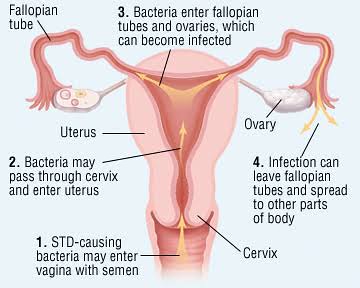The image is an animated, detailed illustration of the female reproductive system displayed against a solid white background. The main focus is a light pink and red drawing of the reproductive organs centered on the page. Black text labels various parts of the anatomy: at the very top left, pointing to a squiggly part, is the "fallopian tube"; directly below this is the "uterus"; and then pointing to the lower portion is the "cervix." Further to the right, another label indicates the "ovary," depicted in white and situated at the end of the fallopian tube on the right side.

Accompanying the anatomical drawing, four numbered points describe the progression of an infection: 
1. "STD-causing bacteria may enter vagina with semen," located at the bottom left, explaining initial infection entry.
2. "Bacteria may pass through cervix and enter uterus," situated in the center near the uterus.
3. "Bacteria enter fallopian tubes and ovaries which can become infected," positioned at the middle top of the image near the fallopian tubes.
4. "Infection can leave fallopian tubes and spread to other body parts," found at the bottom right, pointing to the end of the right fallopian tube.

Yellow arrows trace the path of an infection as it moves through the reproductive system, visually connecting the numbered points. The accompanying text clarifies how infections can travel and spread within the female reproductive organs.